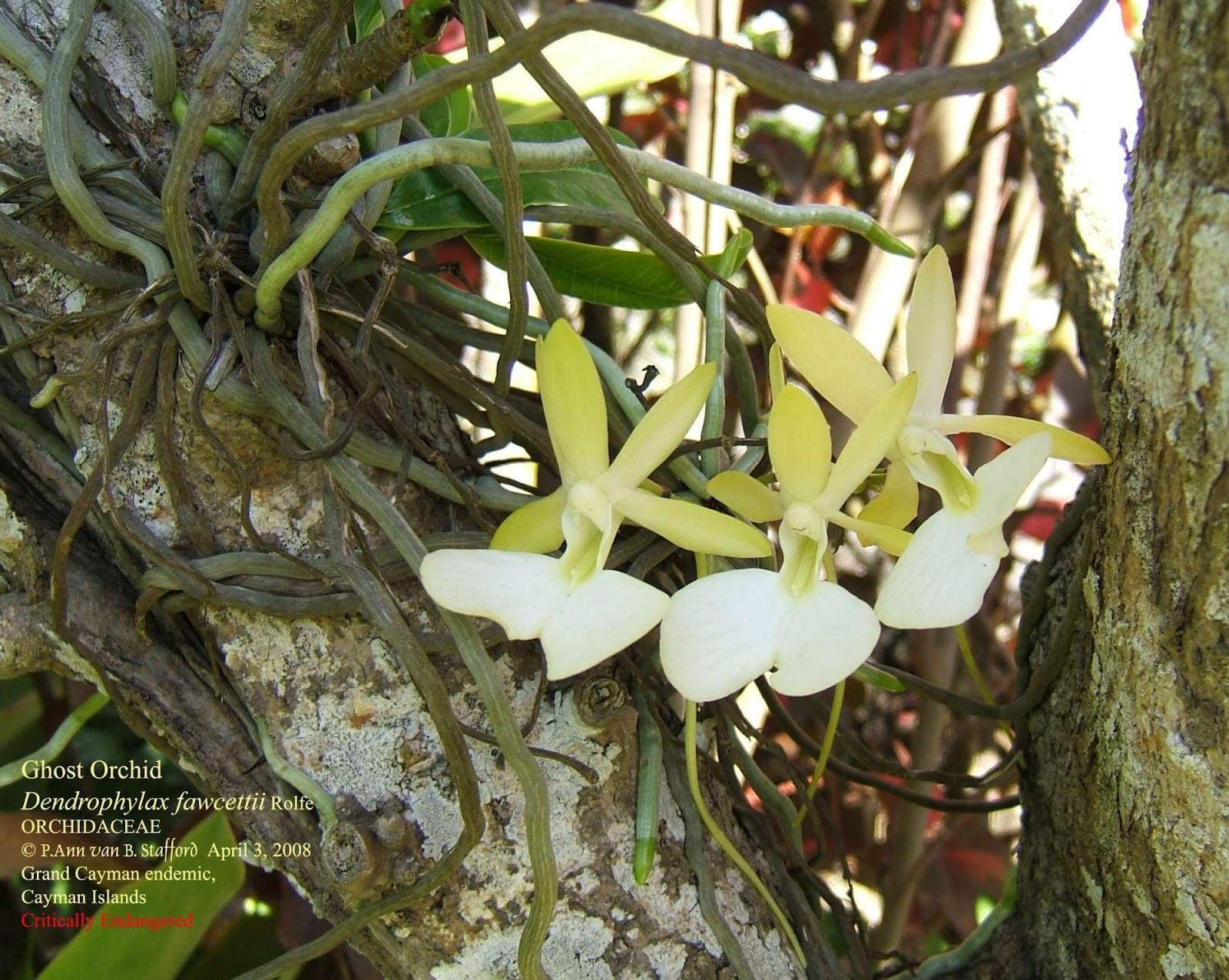The image depicts a close-up photograph of a critically endangered Ghost Orchid (Dendrophylax fawcettii Rolfei) from the Orchidaceae family, endemic to the Cayman Islands. The white and light green star-shaped petals of the orchid are thick and somewhat reminiscent of a green onion. This flower is growing via vines on a large tree trunk, which is visible on the left side of the image along with another vertical tree trunk on the right side. The background features additional vines and plant stems, along with some whitish fungal growth on the tree. In the bottom left corner of the image, yellow text reads, "Ghost Orchid," followed by "Dendrophylax fawcettii Rolfei," "Orchidaceae," and a copyright mark: "© P. Ann Van B. Stafford, April 3, 2008." Below that, it indicates "Grand Cayman Endemic, Cayman Islands," and in red text, "Critically Endangered."